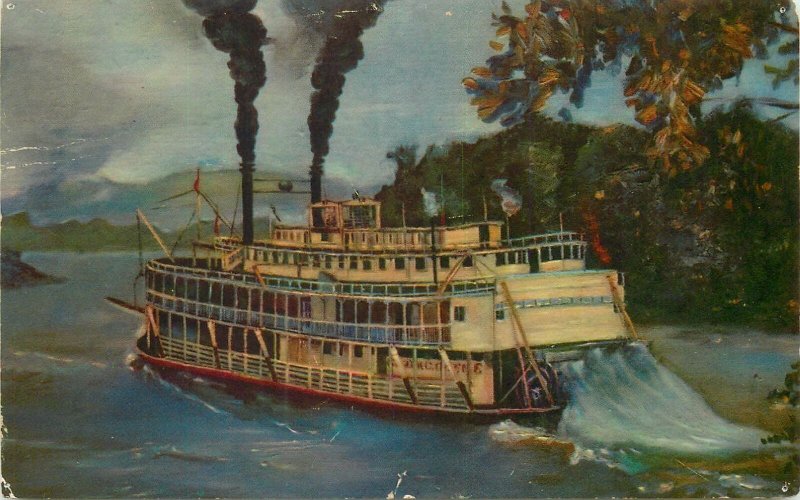This detailed painting on canvas depicts a serene outdoor environment featuring an intricately designed, three-level steamboat navigating through a body of water, possibly a river or canal. The steamboat, which resembles a ferry, has a white structure with a red bottom and distinct water wheels at the back that propel it forward, creating waves. The main deck is open with a balcony, while the second floor houses rooms and the water-level deck is likely the crew area.

Behind the boat, two black smokestacks emit dark clouds of smoke into the sky. The sky itself is light blue with patches of soft gray clouds. The surrounding landscape includes a dense forest of dark green trees on the right side, and in the distance, green hills and a mountainous range add depth to the scene. The canvas retains some imperfections, such as holes, adding a rustic touch to the otherwise picturesque nature setting.